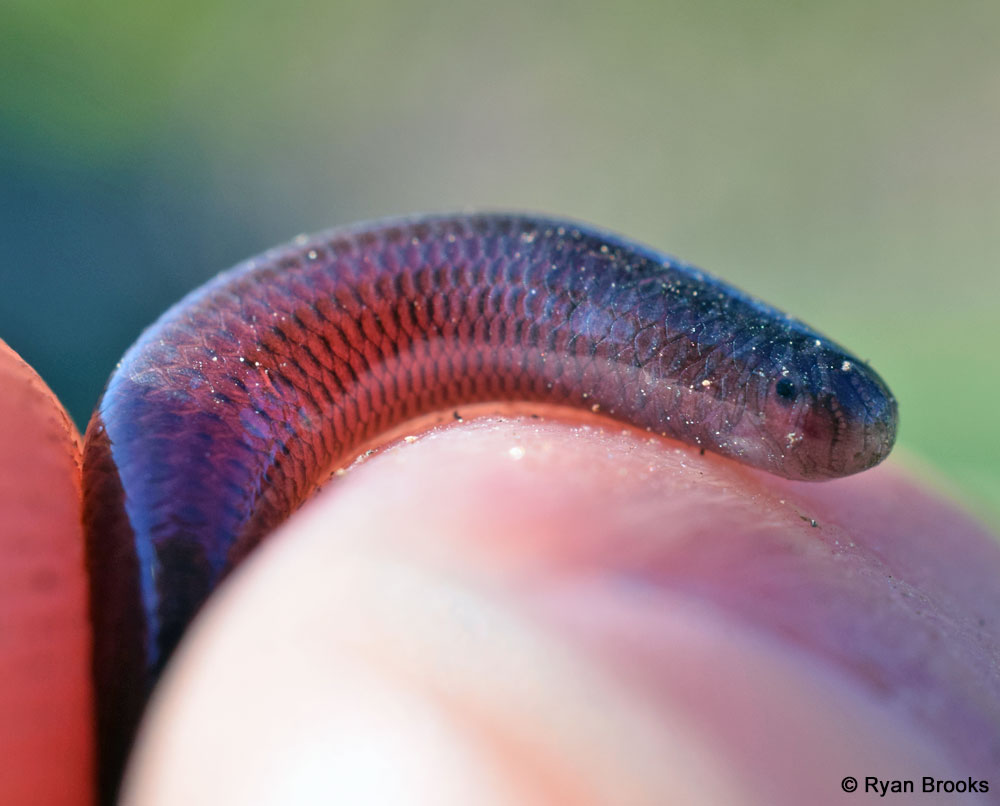This is a detailed close-up photograph, copyright Ryan Brooks, depicting a small, opalescent, iridescent creature, possibly a snake or a worm, being gently grasped between the thumb and finger of a human hand. The creature's skin shimmers with an array of translucent reds, blues, and purples, giving it an almost jewel-like appearance. Its small, rounded face, marked by a single visible black eye, peers outward from its shiny scales that are outlined in black. The head of the creature rests on a fingernail, highlighting its minuscule size. The background is a blurred gradient of green and teal, suggesting an outdoor setting without drawing attention away from the main subject. The overall image is dynamic yet serene, capturing the delicate beauty and mysterious nature of this tiny, radiant animal in exquisite detail.